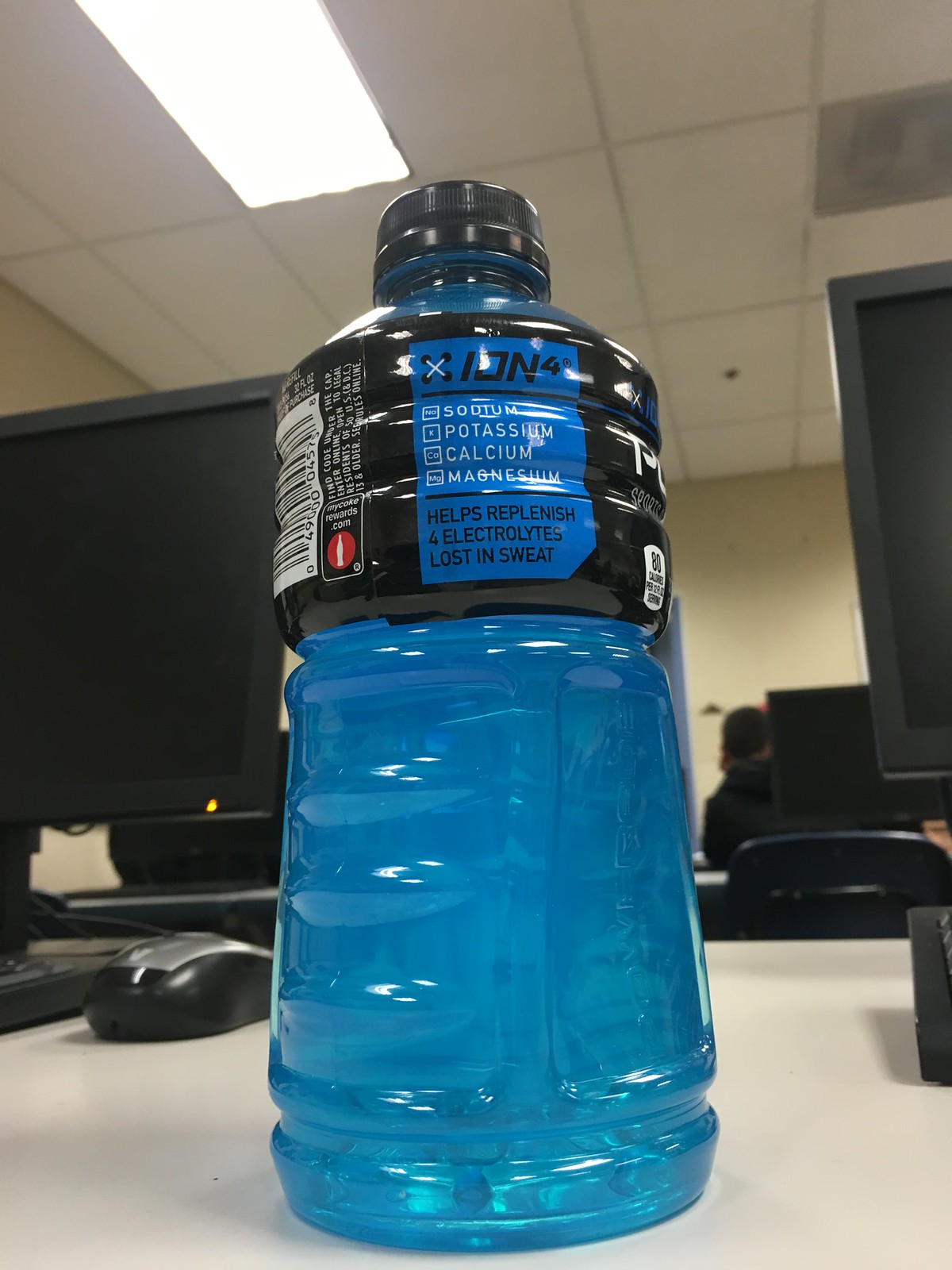A pristine, full bottle of an electrolyte drink sits prominently on an immaculate white desk in a modern office setting. The sleek, black label covers the top half of the bottle, featuring "X-ion-4" in bold lettering, and lists sodium, potassium, calcium, and magnesium as key ingredients. Below, the text reads, "helps replenish four electrolytes lost in sweat." The bottle cap is also black, complementing the label. The light blue liquid inside contrasts sharply with the monochrome office environment. In the background, rows of identical desks and chairs are accompanied by turned-off computer monitors. The office is mostly empty, save for a man with black hair, donned in a black hoodie, working at a computer against the opposite wall. The scene captures a moment of stillness amidst a typically bustling workspace.